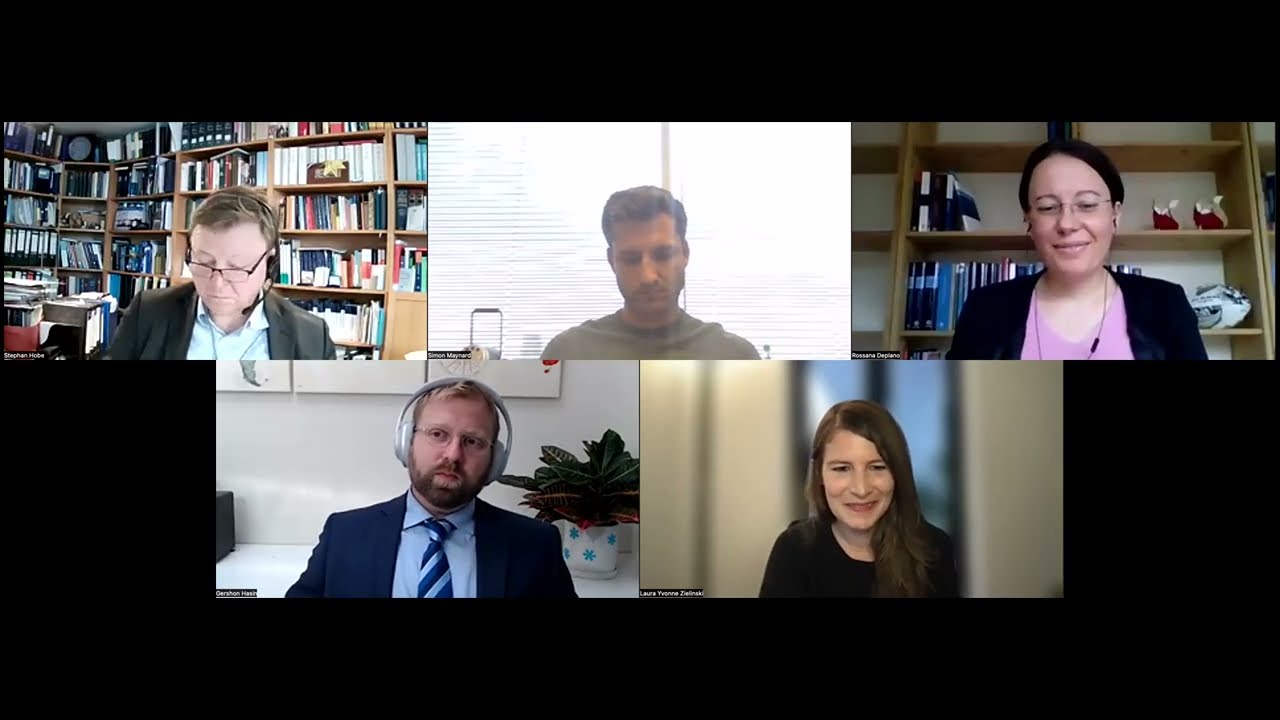This image captures a Zoom meeting featuring five participants, arranged in a grid with three people on the top row and two on the bottom. The top left shows a man wearing glasses and a gray and blue outfit, looking down, with a giant bookshelf behind him. In the center top position is another man framed by a backdrop of glaring windows, also looking down. To the top right is a woman wearing glasses, dressed in dark blue and pink, smiling in front of a tidy bookshelf. On the bottom row, the left image includes a man in a blue suit with gray headphones, accompanied by a potted plant beside him. Finally, the bottom right image features a woman with long brown hair, smiling, against a blurred background. The overall layout is clear and well-organized, representing a typical video call session on platforms like Skype or Zoom. The image's colors include black, brown, blue, gray, pink, purple, and white, framed by black borders at the top and bottom.